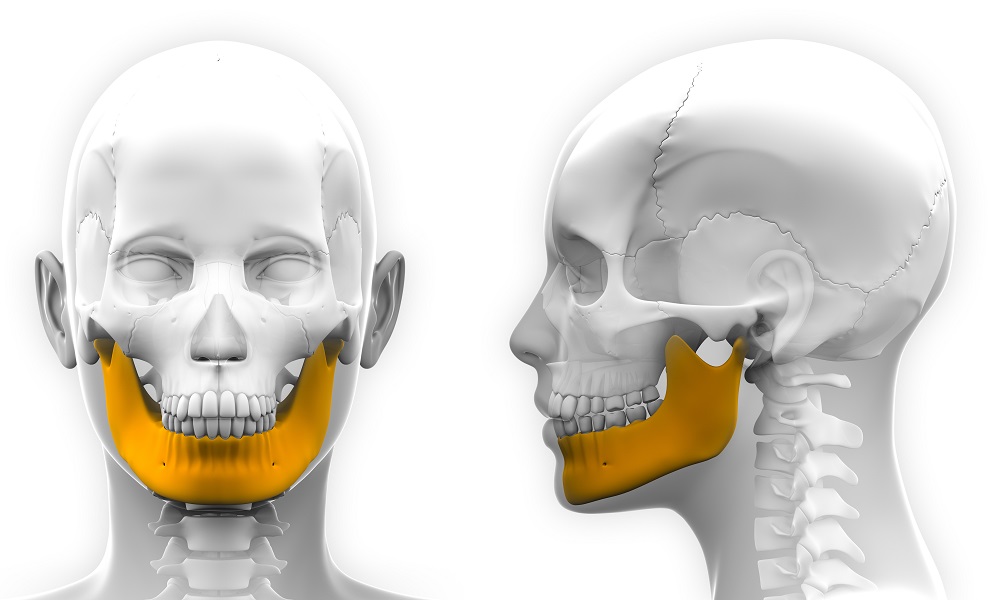The image features two artistically rendered, semi-transparent human skulls, depicted in a grayscale. The skull on the right faces directly toward the camera, revealing the front of the face. Its top is primarily white with subtle gray shading around the eyes and along the sides. The eye sockets themselves are white, while the nose and ear are rendered in a darker gray. The jawline is white, but the lower jaw or mandible is highlighted in a golden-orange hue, which also shows off the white teeth. Below the jawline, the white spine and neck outline are discernible.

The second skull is the same as the first but shown in profile, facing left with the back of the head on the right side. This skull maintains the white color scheme with similar gray shading, including a dark eye socket and the side of the nose. Like the first skull, the jawline is white, with the lower jaw highlighted in the same golden-orange color, displaying the white teeth clearly. The spine is also visible below the skull, rendered in white and highlighted through the semi-transparency of the neck.

The entire image has a textbook or illustrative feel, possibly designed for educational purposes like an anatomy presentation. The background is white, enhancing the grayscale and highlighted features of the skulls. The depiction includes visible natural fissures and the top seven vertebrae, emphasizing anatomical details while maintaining a clean, computer-generated 3D appearance.